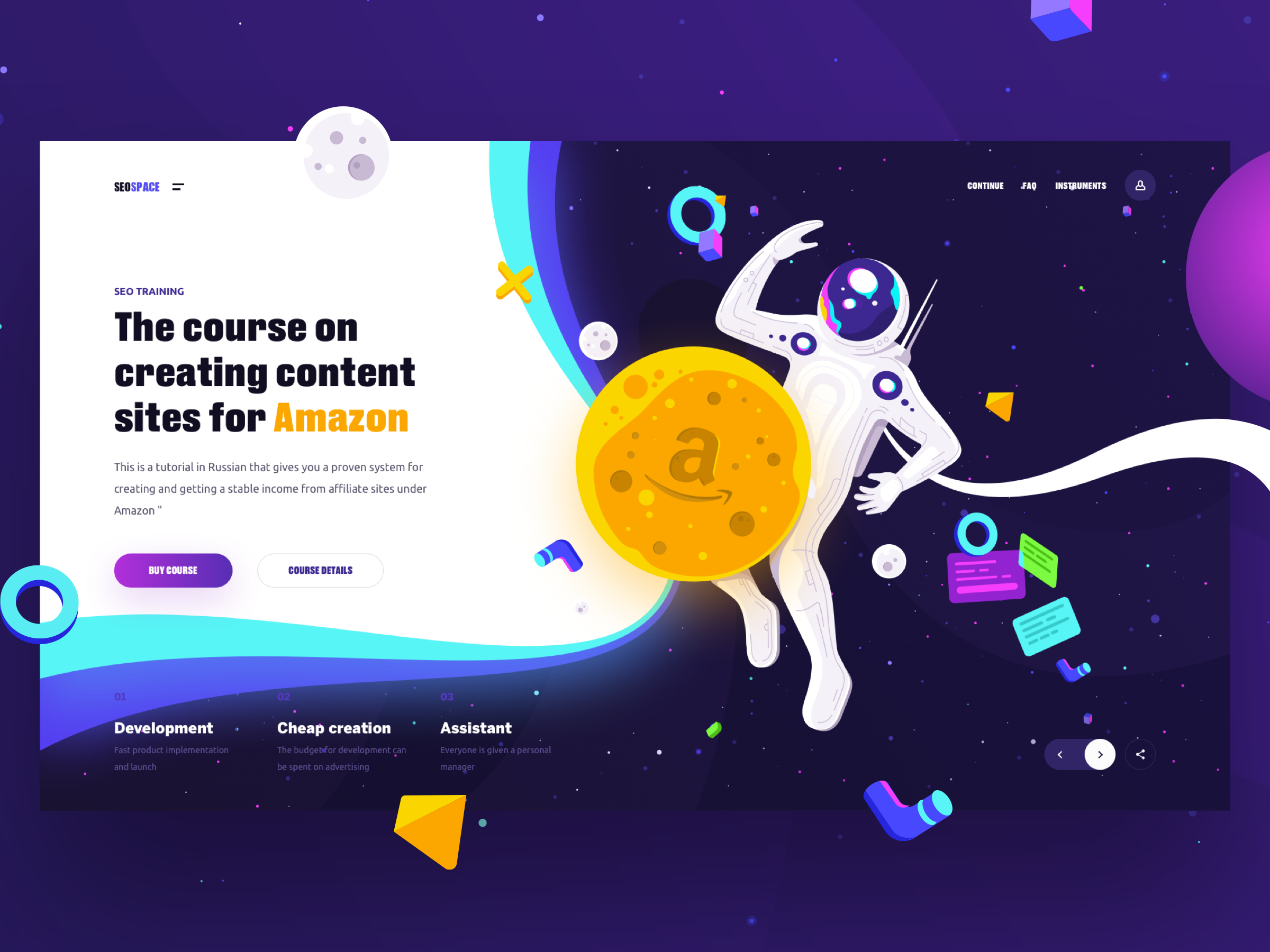Header image showcasing a vibrant and playful portfolio page designed with a space theme. The background is a lively array of purple hues interspersed with various shapes in shades of blue, green, and orange, creating a whimsical, cartoon-like aesthetic. Central to the image is a screencap of a website dedicated to SEO training, titled "SEO Training: The Course on Creating Content for Sites for Amazon". This tutorial, available in Russian, offers a proven system for achieving stable income through affiliate sites on Amazon.

Below the main course title, there are two buttons: a gradient purple button with white text labeled "Buy Course" and a white button with purple text labeled "Course Details." Further down are three columns labeled "Development," "Sheet Creation," and "Assistant," though the associated descriptive text is too small to discern clearly.

An astronaut is whimsically floating amidst various space-themed elements, adding to the page's dynamic yet minimalistic design. A standout feature is a bright yellow planet with the Amazon logo at its core. The overall layout is easy-going and fluid, characterized by its simple yet intensely colorful and fun art style.